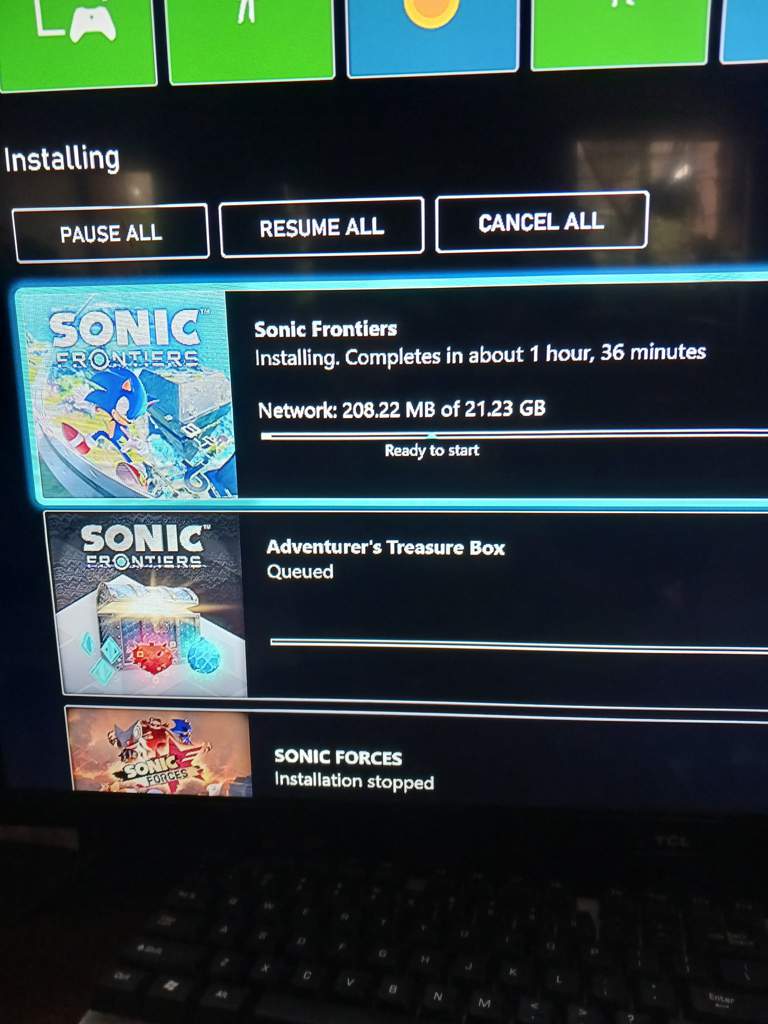A person is working on a Windows laptop, as evidenced by the visible keyboard. The screen displays the Xbox gaming site on the Microsoft Store. The Microsoft Store section is partly cut off but shows five colorful icons at the top: three green and two blue. One blue icon features a sun.

On the left side of the screen, a section marked in white text on a black background indicates that something is currently installing. Below this section, there are three buttons labeled "Pause All," "Resume All," and "Cancel All."

The main image displayed on the screen is the cover artwork for "Sonic Frontiers," showcasing the iconic blue hedgehog. The game is in the process of installing, with details indicating that 208.22 megabytes have been downloaded out of the total 21.23 gigabytes required.

Additionally, thumbnails for "Sonic Frontiers" and "Sonic Forces" are displayed further down. The second "Sonic Frontiers" thumbnail shows no current activity, implying it's not actively being downloaded. Meanwhile, "Sonic Forces" appears to have had its download stopped.